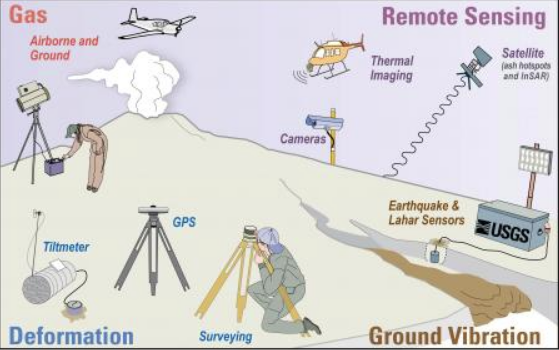An infographic illustration portrays a detailed scene centered around a beige-colored mountain emitting white smoke from its peak. In the upper left corner, red letters spell out "Gas, Airborne, and Ground," situated slightly to the side of the smoke plume. Dominating the sky above the mountain, a gray, single-prop airplane flies overhead, symbolizing aerial observation. 

On the ground, various personnel and equipment are actively engaged in monitoring and surveying activities. A woman is seen bending over a purple box, adjusting an instrument positioned atop it, suggesting the use of specialized observation equipment. Other surveyors are depicted looking through lenses mounted on numerous tripods, which are colored in shades of yellow and gray. These tripods appear to hold various meters and instruments essential for environmental measurements.

Additionally, a gray surveillance camera perched on a yellow post is marked with the label "Cameras." The top right corner of the infographic highlights "Remote Sensing," and includes an illustration of an orange helicopter equipped with a sensor, denoted by a Wi-Fi icon-like graphic emanating from its bottom.

A depiction of a satellite with a wavy line extending downwards illustrates thermal imaging capabilities. Additional information is presented alongside this graphic, further emphasizing the comprehensive data collection. On the far right of the image, a gray box labeled "USGS" (United States Geological Survey) stands out, accompanied by a standing light or another type of lighting device overhead. This informative visualization captures the extensive measures taken for geological monitoring and data collection.